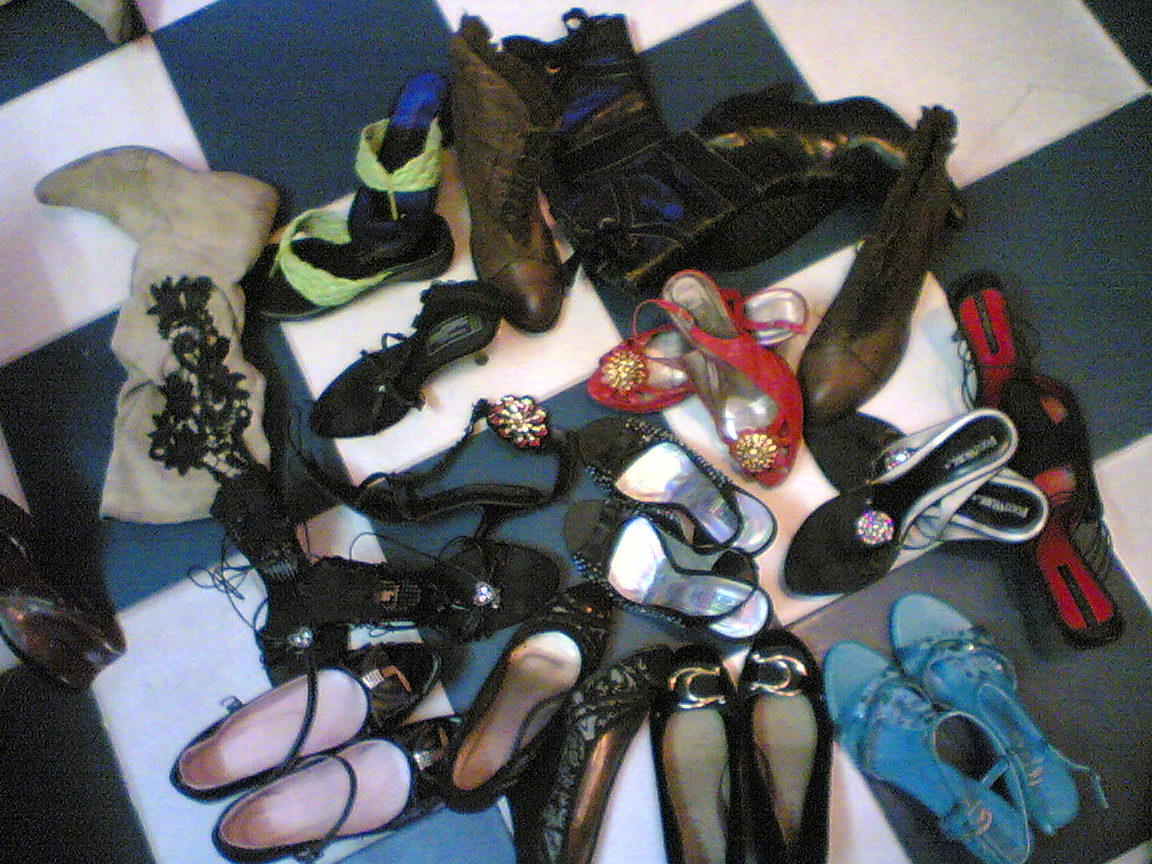In this photograph taken from above, a diverse collection of women's shoes is scattered across a black-and-white vinyl checkered floor. The assortment includes a variety of high heels, boots, flats, and slip-on shoes in multiple colors and styles. Notable footwear among the pile includes red pumps centrally positioned, light blue heels in the bottom right corner, and a pair of old beige suede boots in the top left. Black shoes dominate the scene, featuring black flats, black high heels, and black leather boots. There are also brown cowboy boots, brown combat boots, black cowboy boots, and a mix of heels adorned with straps or designed to be slipped on. The overall arrangement of the shoes is haphazard and messy, adding a casual and spontaneous feel to the image.